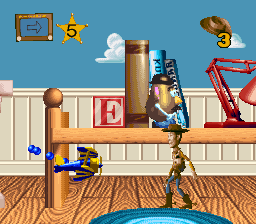In this vibrant still image from a Toy Story-themed video game, we find ourselves in a lively, animated room reminiscent of a child's bedroom. The wooden floor and a matching wooden desk dominate the scene, complemented by a blue round rug with varying shades of blue. Woody, the iconic cowboy from Toy Story, stands by the rug, adorned in his signature vest, cowboy boots, and cowboy hat. 

On the desk, there are three vertically standing books, a red lamp, and an alphabet block showcasing the letter "E". Mr. Potato Head is positioned in front of the books. The playful decor extends to the walls, which feature a blue paint job decorated with fluffy cloud designs and white batten board trim. High on the wall, an Etch-A-Sketch displays an arrow, while a brown cowboy hat marked with a '3' and a sheriff star with the number '5' are also visible. Additionally, a blue and yellow toy airplane flies around the scene, adding a whimsical touch to the immersive environment.